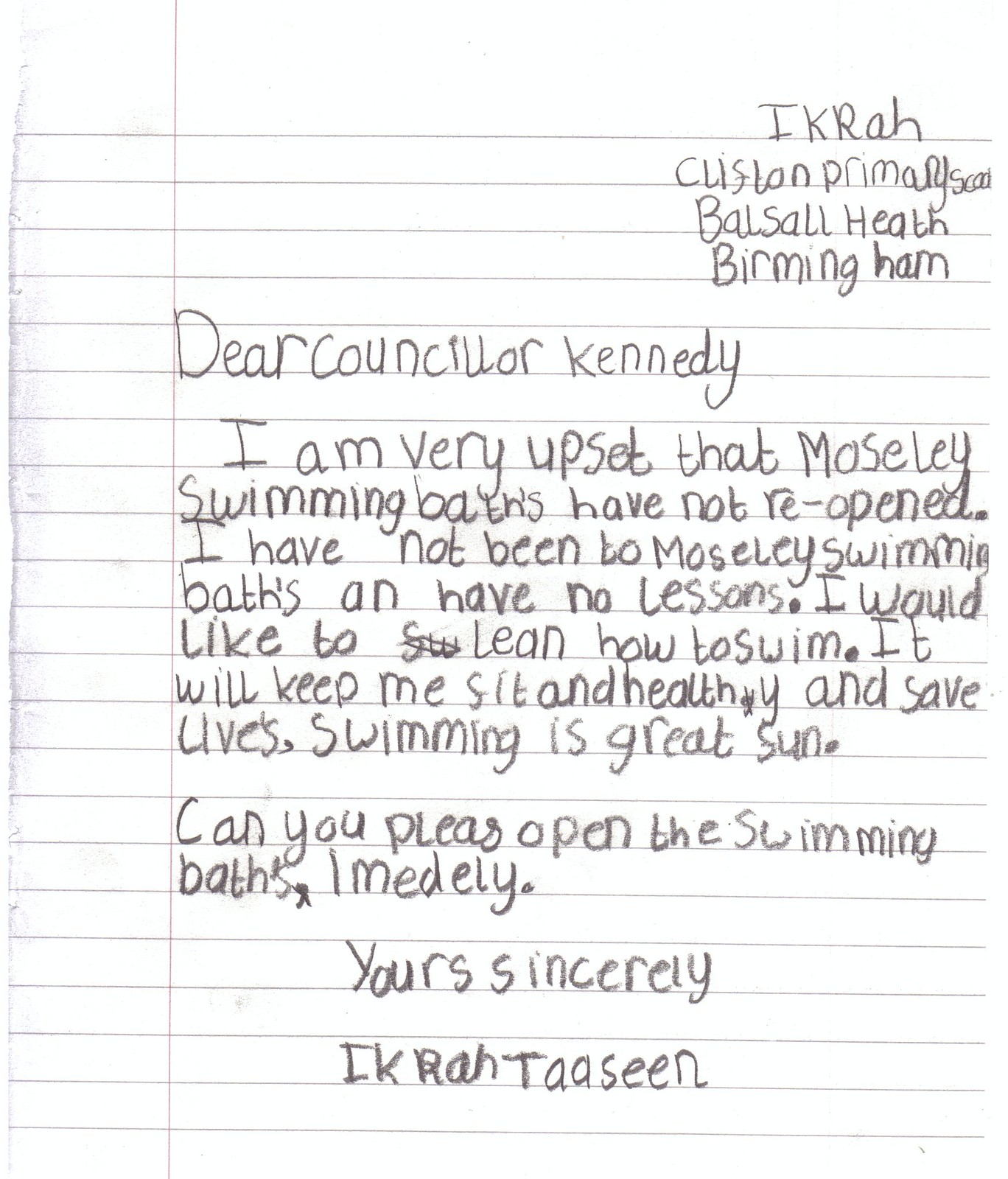The image depicts a scan of a handwritten letter on a lined page torn from a notebook. The writing, which appears unsteady as if written in pencil, includes a header in the upper right corner that reads, “Ikrach Klichon Primary School, Balzau Heights, Birmingham.” The body of the letter, addressed to Councillor Kennedy, expresses the writer's distress over the ongoing closure of the Mosley Swimming Baths. The letter states:

“Dear Councillor Kennedy,

I am very upset that Mosley Swimming Baths have not reopened. I have not been to Mosley Swimming Baths and have no lessons. I would like to learn how to swim. It will keep me fit and healthy and save lives. Swimming is great fun. Can you please open the swimming baths immediately?

Yours sincerely,
Ikrach Tassin”

The letter conveys a heartfelt appeal for the reopening of the local swimming facility, emphasizing its importance for physical fitness, safety, and enjoyment.